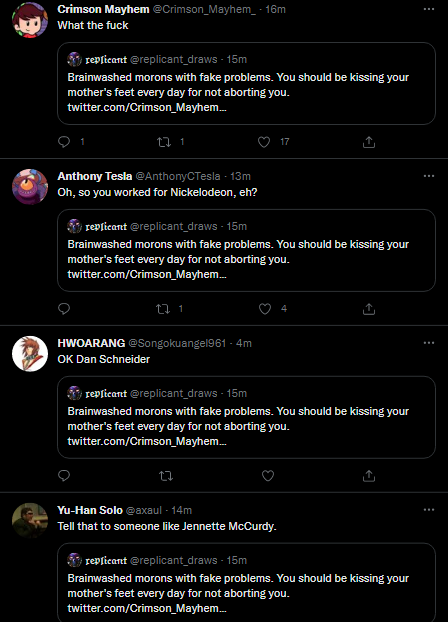**Screenshot of a Heated Twitter Exchange**

The image is a screenshot of a Twitter chat, featuring a controversial tweet from the user "Crimsome Mayhem" with the handle @crimsome_mayhem_. The tweet, posted 16 minutes ago, reads: "You replicant brainwashed morons with fake problems. You should be kissing your mother's feet every day for not aborting you." This message is accompanied by a link to the tweet on twitter.com.

In response, "Anthony Testa" @tesla replied with, "Oh, so you work for Nickelodeon?" alongside a question mark. The original tweet's offensive message is echoed multiple times in the conversation thread.

Another user, "Hwoarang" (@Hwoarang), also reiterated the same disrespectful tweet: "You replicant brainwashed morons with fake problems. You should be kissing your mother's feet every day for not aborting you," including a link to Crimsome Mayhem's tweet.

Lastly, "Yuhan Solo" @Yuhan_Solo adds to the exchange with the remark, "Tell that to someone like Janet McCordie," followed once again by the repeated text: "You replicant brainwashed morons with fake problems." 

The screenshot captures a snapshot of a hostile discussion on Twitter, highlighting the repetitive derogatory remarks and the ensuing reactions from different users.